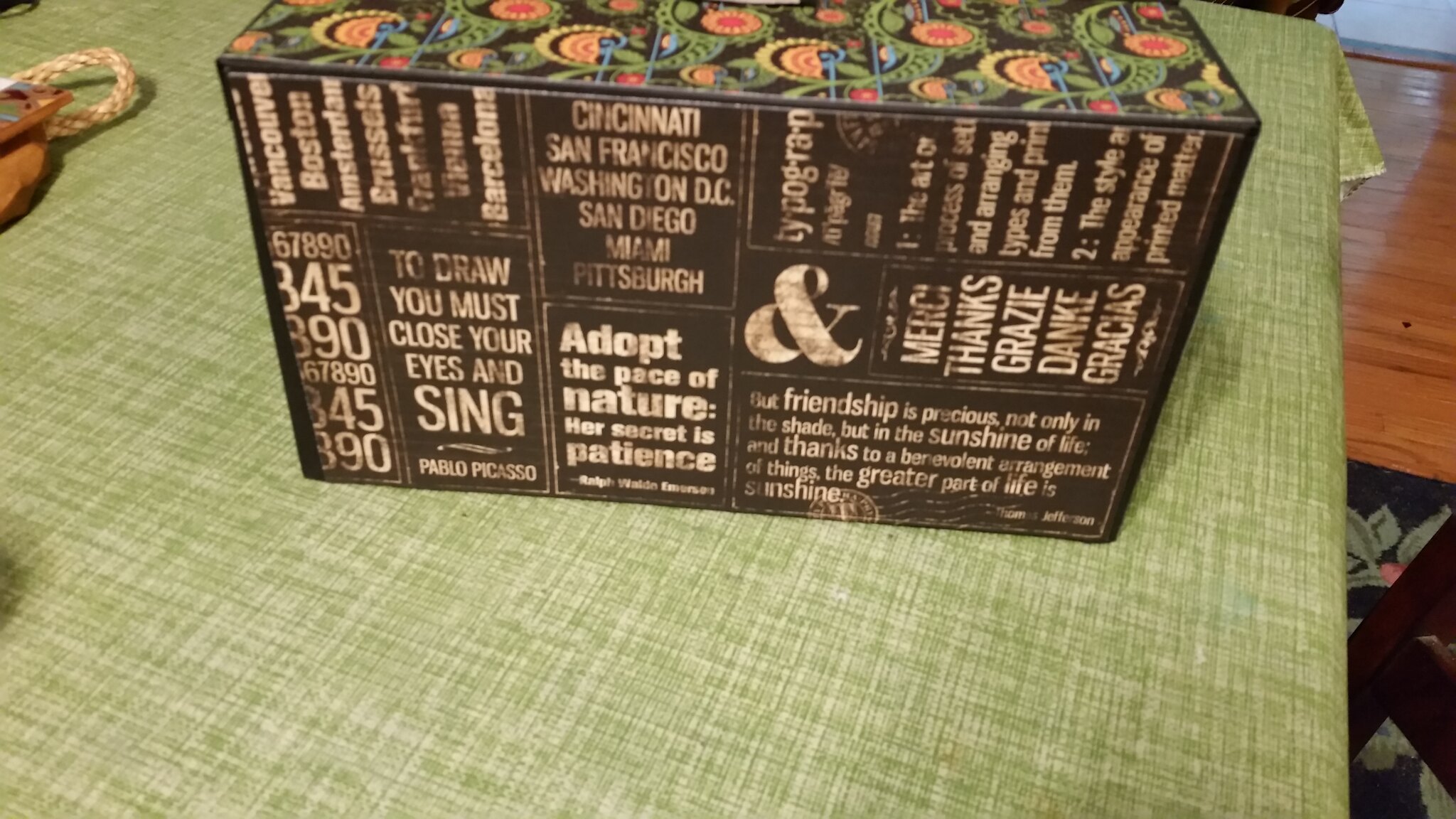The photograph captures a detailed view of a central box placed on a green and white tablecloth. The box, predominantly brown, features a top adorned with colorful patterns including orange, blue, and green floral paisley designs. The front-facing side is black with worn cream-colored writing and an assortment of texts. Notable inscriptions include phrases such as "Adopt the pace of nature. Her secret is patience," "To draw, you must close your eyes and sing," "Merci, thanks, grazie, danke, gracias," and city names like "Cincinnati, San Francisco, Washington D.C., San Diego, Miami, Pittsburgh." Quotes from various individuals, including Pablo Picasso and Thomas Jefferson, are also present, along with a large ampersand symbol. In the background, a reddish-brown wooden bench or structure is visible, adding depth to the image, while the table's light green tablecloth complements the intricate design and vibrant colors of the box. The overall setting provides a visually rich composition with a blend of textual detail and colorful embellishments.